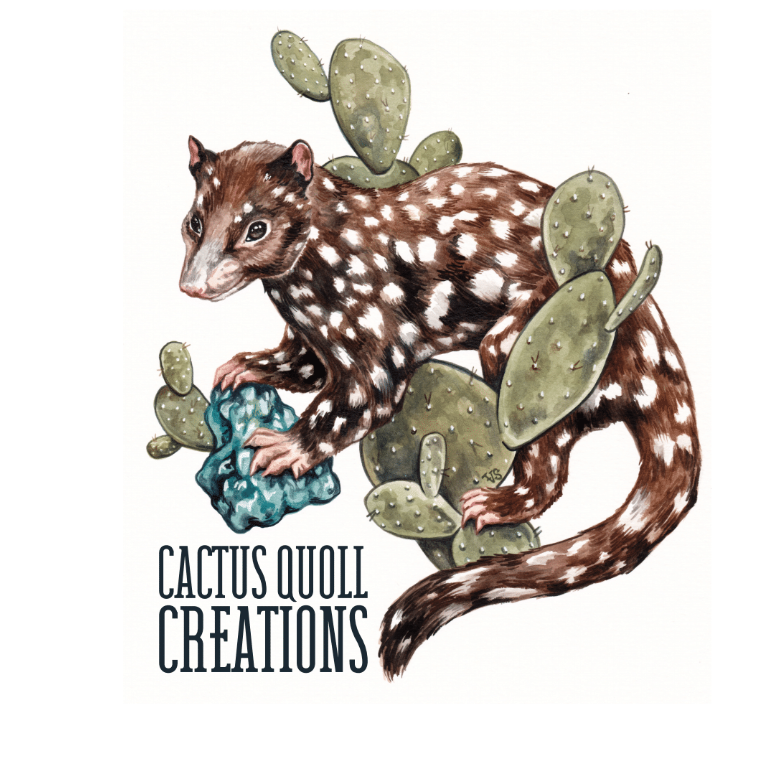This is a detailed illustration, possibly created with watercolor or pen and ink, featuring a desert animal and a cactus set against a plain white background. In the bottom left corner, it is signed "Cactus Quoll Creations." The depicted animal resembles a quoll, characterized by its black fur with white polka dot-like spots, a long tail, short ears, and a elongated snout. The creature stands amidst a large, flat green cactus with typical spiky edges. Notably, the animal holds an aqua-colored object with white highlights, possibly a stone or cloth, between its front paws. The illustration captures the essence of a desert scene with a focus on the contrasting elements of the dark-spotted animal and the vibrant green cactus.